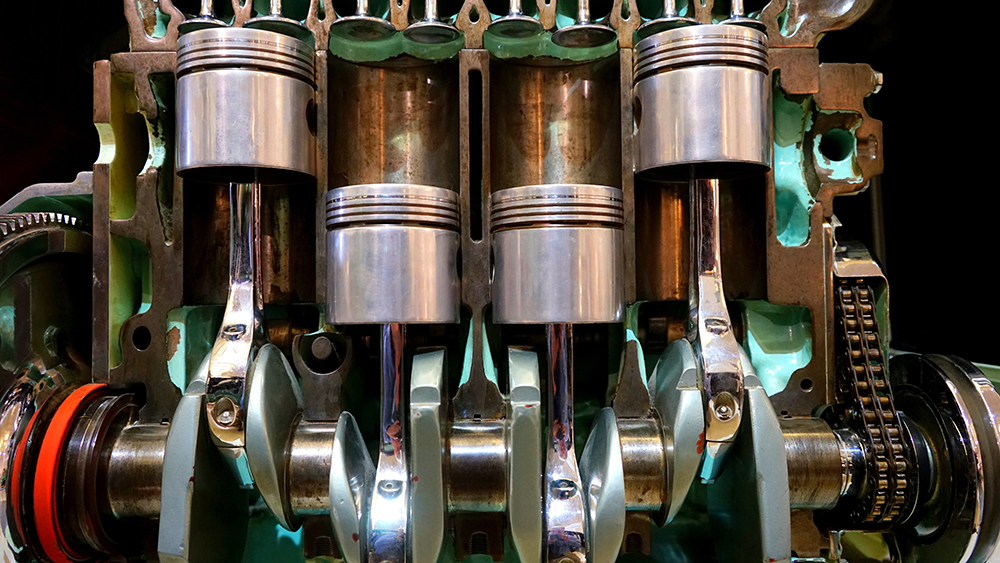The image depicts a detailed cutaway view of a four-cylinder engine, showcasing various mechanical components primarily made of metal, including steel, aluminum, and possibly copper. The engine features four pistons housed in separate cylinders, with the outer two pistons in the up position and the inner two in the down position. There are several chains and belts integrated into the design, with a notable red belt wrapped around some levers on the left side. The engine includes multiple gauges, valves, and plugs that facilitate its operation, as well as a cylindrical axis at the bottom terminating in two wheel-like endings, one of which has a distinctive red stripe. The overall object appears well-maintained and exhibits a range of colors from light green to discolored copper tones, giving an impression of a well-used but functional piece of machinery. This intricate setup is likely intended for industrial or automotive use, situated indoors, as suggested by the upright orientation and the presence of oil around the chains.